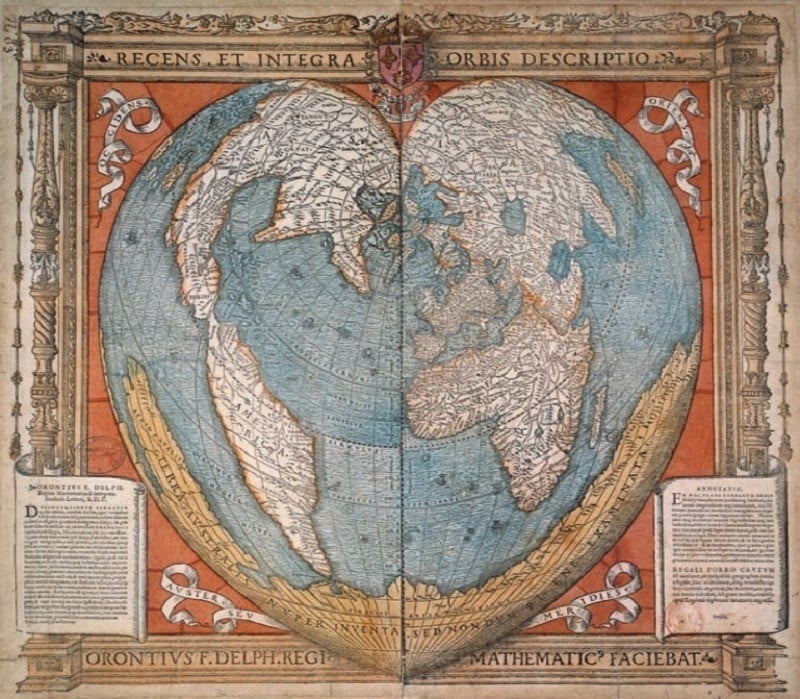This photograph appears to be from an old text, showcasing a fascinating world map depicted in a unique heart-shaped design. The map is illustrated across two pages with a central fold, prominently featuring the continents—North and South America, Europe, Asia, and Africa. At the top, the Latin title "Recens et Integra Orbis Descriptio" translates to "Recent and Complete Description of the World." Stone pillars in gray and tan encase the map, adorned with additional Latin inscriptions, one of which mentions "Mathematic," hinting at mathematical undertones in the cartography. A ribbon beneath the globe holds more Latin text, including "ORONTIVS F.DELPH.REGI Mathematica FACIEBAT," suggesting an attribution to Orontius and emphasizing the mathematical crafting of the map. The bottom portion also alludes to "Terra Australis Incognita," believed to be the then-mysterious southern landmass, indicative of the era’s geographical theories. The ornate framing and classical elements, combined with the ancient Latin script, suggest this artifact could date back to the 16th or 17th century.